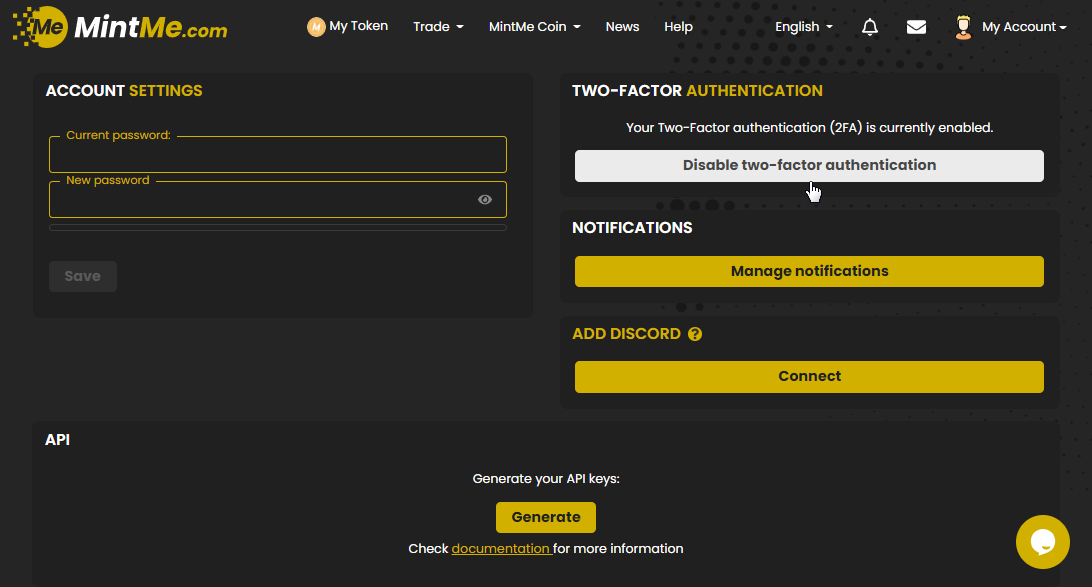On the top left of the image, the text "mintme.com" is displayed, where "mint" is in white and "me.com" is in yellow. To the left of the name, there is an orange circular icon with the letters "ME" written inside. Yellow squares are arranged sequentially from the center of the circle extending to both the right and left sides. 

Along the top of the page are several tabs labeled "My Token," "Trade," "Mint Me Coin," "News," "Help," and "English." Additionally, there are icons for notifications, inbox, and user account on the top right. The user avatar is a blend of yellow and orange.

The background of the entire page is blank. On the left side, the text "Account Settings" is displayed, where "Account" is in white and "Settings" is in yellow. Below this are two fields outlined in yellow: "Current Password" and "New Password," both featuring yellow text. There is a gray "Save" button below these fields.

On the right side, the text "Two-Factor Authentication" is presented, with "Authentication" highlighted in yellow and "Two-Factor" in white. It mentions that 2FA is currently enabled. There is a white button with black text labeled "Disable Two-Factor Authentication." Below this section, there is another labeled "Manage Notification," featuring a yellow button with black text reading "Connect." Further down, a small text prompts "Add Discord," accompanied by a yellow button with black text that says "Connect."

At the bottom on the left, the label "API" is visible, with "Generate your API keys" in the center. There is a yellow button below this text saying "Generate." Further instructions to "Check documentation for more information" are noted below.

In the bottom right corner, there is a white circular icon with a speech bubble outlined in yellow, designated for assistance.